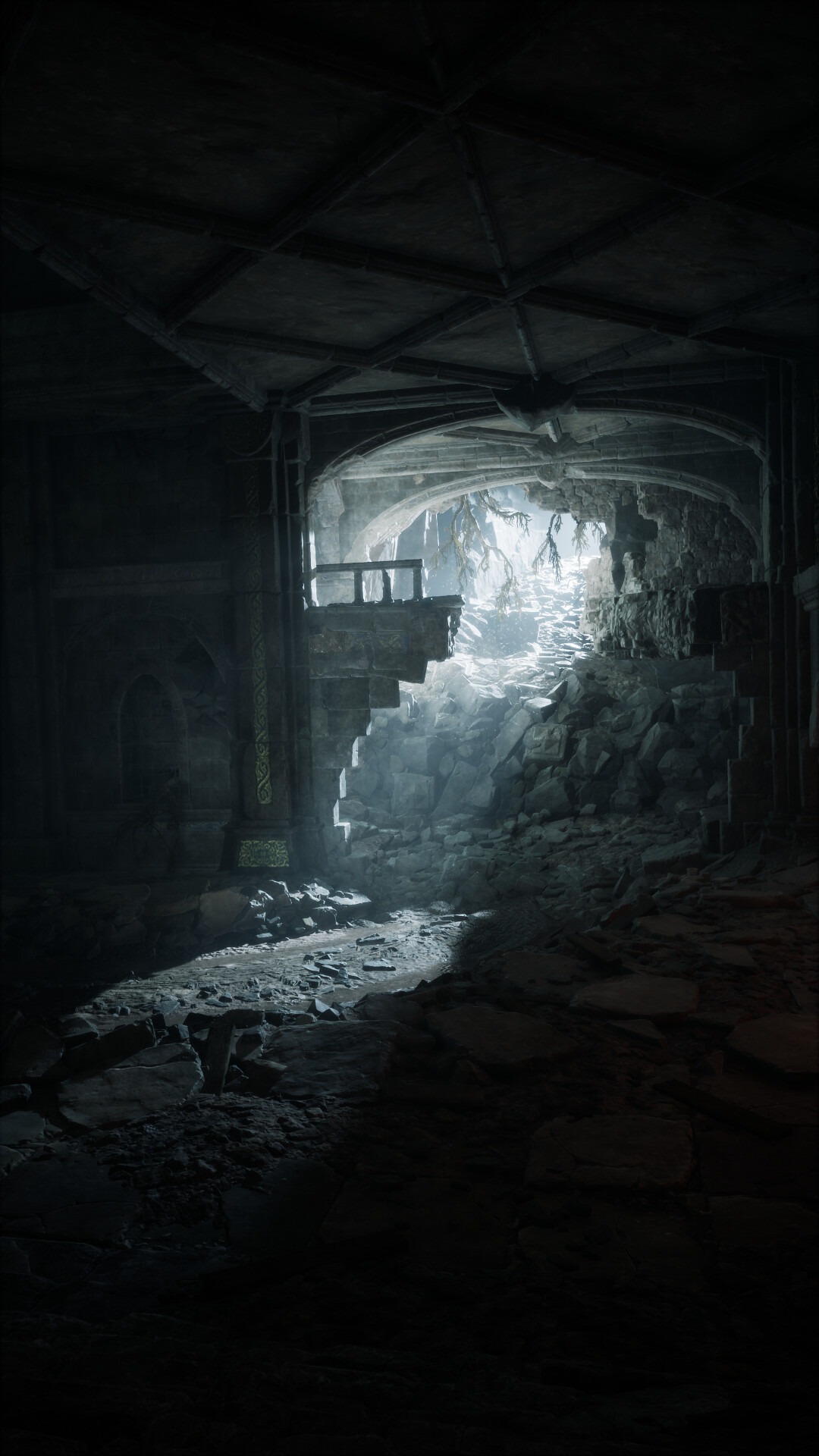A screenshot, likely from a video game, depicts the interior of an abandoned building with a rough stone floor. The room features an arched doorway, partially demolished, revealing remnants of the old blocks that once supported the structure. The ceiling is supported by rough wooden beams, adding to the dilapidated atmosphere. Through the doorway, a rocky path extends into the distance, illuminated by daylight and leading towards a forested area. The stark contrast between the dark, shadowy interior and the bright, inviting exterior emphasizes the building's state of decay and abandonment.